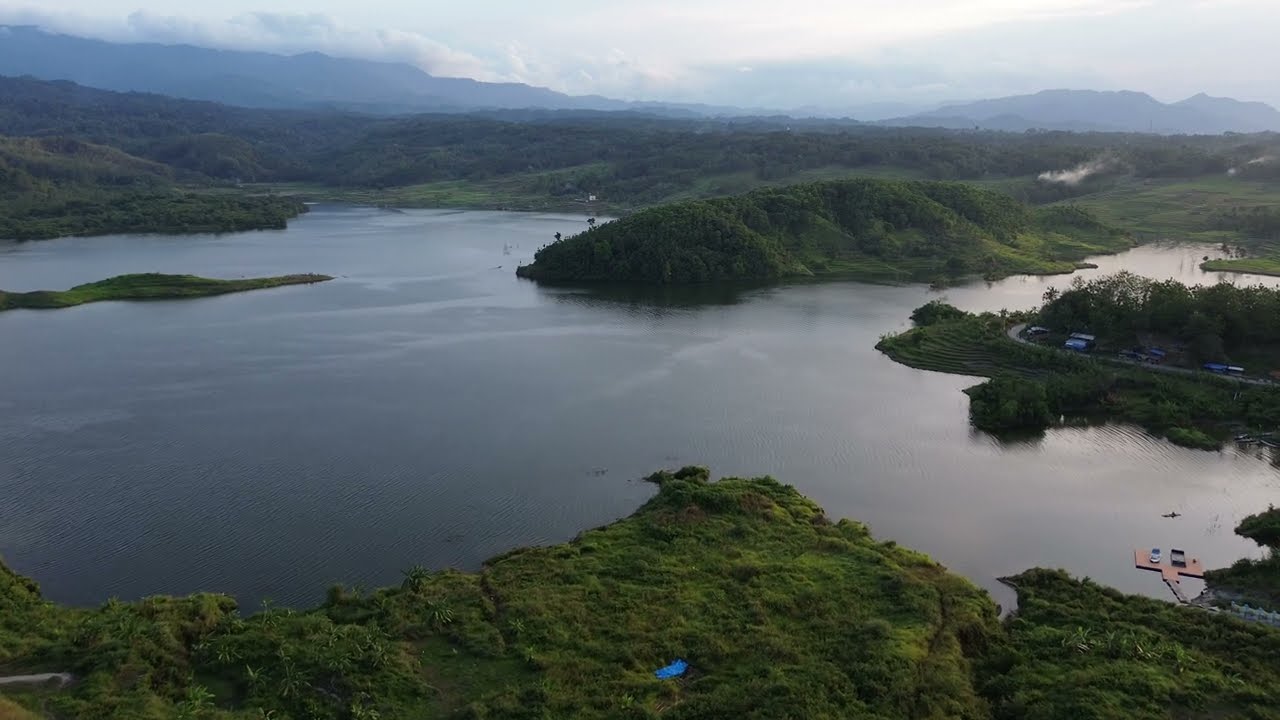This is an aerial view capturing a vast lake landscape. In the far background, a range of mountains and hills are being gently embraced by clouds, giving a sense of haziness and fog. The sky above is a mix of white clouds and light blue patches. The landscape is predominantly green, with mountains and hills covered in lush greenery like trees and grass. 

The lake itself is a serene expanse of blue and gray water, noticeable for its calmness and lack of any visible boats or waves, making it almost reflective. On the right side of the image, a tan-colored dock extends out onto the placid water. There is also a prominent piece of land jutting into the lake on the right, which features a road and several blue and brown squared and rectangular-shaped buildings. In addition, the lake is bordered by more shoreline that appears to narrow but isn't fully visible on the left. The overall scene conveys a tranquil and picturesque natural environment.